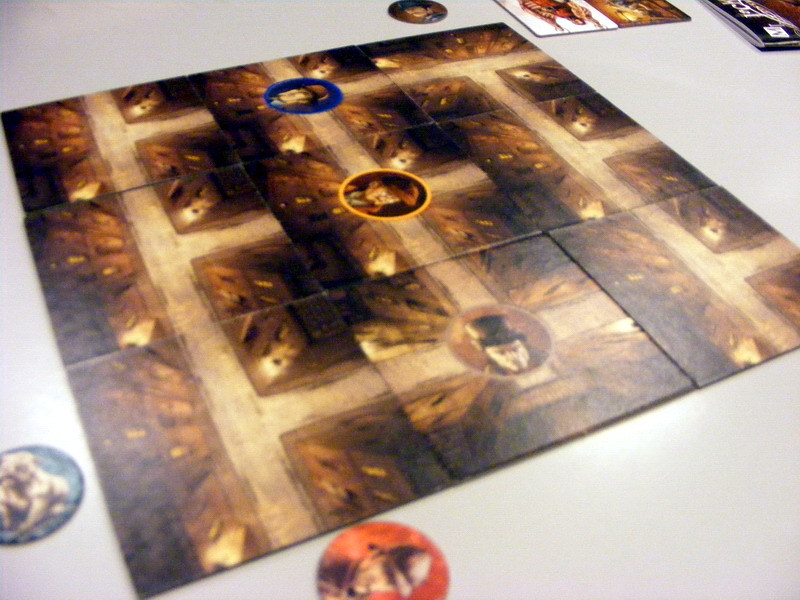The image depicts a white table featuring a board game with a 3x3 grid of squares, reminiscent of a tic-tac-toe layout. Each square houses a circle, three of which prominently display the faces of gentlemen donning various hats. The top circle has a blue outline, the middle a yellow outline, and the bottom a white outline. At the table's edge lies a circular token with a red background, featuring another hat-clad man. To its left is a blue-bordered token displaying a dog, while an additional token with a man in a black hat is positioned in the upper middle part of the photo. Beside these tokens rest two square cards with indiscernible images. Partially peeking into the frame is a magazine, adding to the array of objects on the table. The setup includes abstract and colorful elements, giving the scene an artistic flair.